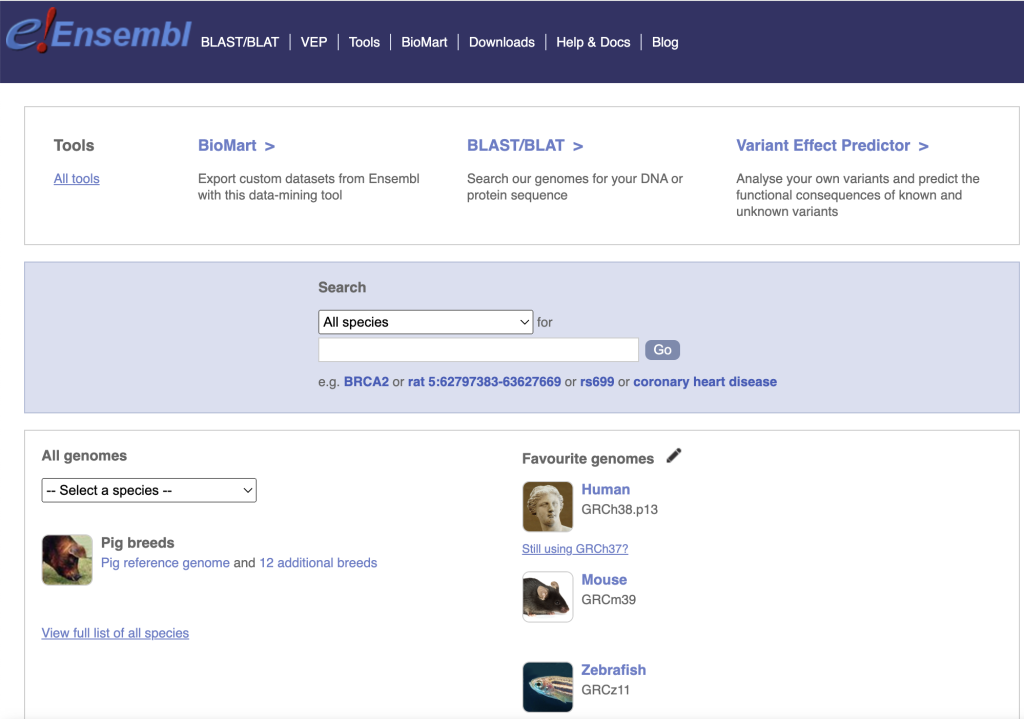This image is a screenshot taken in landscape mode, likely from a laptop. It displays a webpage with a structured layout. 

At the very top, there is a dark blue banner spanning from the upper left corner to the upper right corner. On the far left of this banner is a logo, showcasing the capital letter "E" followed by a red exclamation point, spelling "ENSEMBL."

Directly to the right of the logo, a series of tabs are arranged horizontally. These tabs read as follows: "Blast," "Blat," "VEP," "Tools," "Biomart," "Downloads," "Help and Docs," and "Blog."

Beneath the dark blue banner, the next row features a white background and is divided into four distinct columns. The first column is labeled "Tools," with the text "All Tools" underlined in blue. Below this, it reads, "Biomart" in blue, followed by the descriptive text, "Export custom data sets from Ensembl with this data mining tool."

The second column is labeled "Blast," followed by "Blat" in blue text beneath it, accompanied by the text, "Search our genomes for your DNA or protein sequence." The third column features "Variant Effect Predictor" in blue, with the explanatory text, "Analyze your own variants and predict the functional consequences of known and unknown variants."

Following this, there is a row with a light gray background. The text in this row reads, "Search all species."

The subsequent row features a white background with two main columns. The left column is titled "All Genomes" and includes a dropdown labeled "Select a species," followed by the text "pig breeds." Below this, there is a link that reads, "View full list of species."

In the right column, the title "Favorite Genomes" is displayed, listing "Human," "Mouse," and "Zebrafish" with small thumbnail images next to each genome.

This detailed layout offers a comprehensive view of the webpage, highlighting the navigational elements and main functional areas.